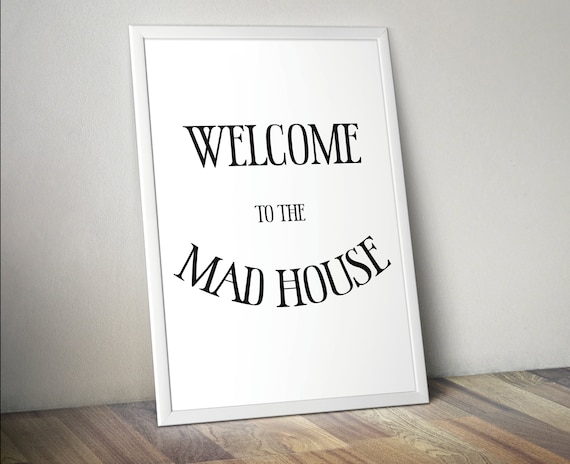The image captures a framed poster propped against a gray wall on a wood floor with visible grains and a mix of tans and darker browns. The frame is white and narrow, encapsulating a white background. The poster features black, capitalized lettering. At the top, the word "WELCOME" is prominently displayed in a straight line. Below it, in slightly smaller uppercase letters, it reads "TO THE." At the bottom, the word "MADHOUSE" is written in a black font and is curved in an upward arc, reminiscent of a smile. The overall visual effect is a simple yet bold textual design that draws attention with its clear, monochromatic contrast.